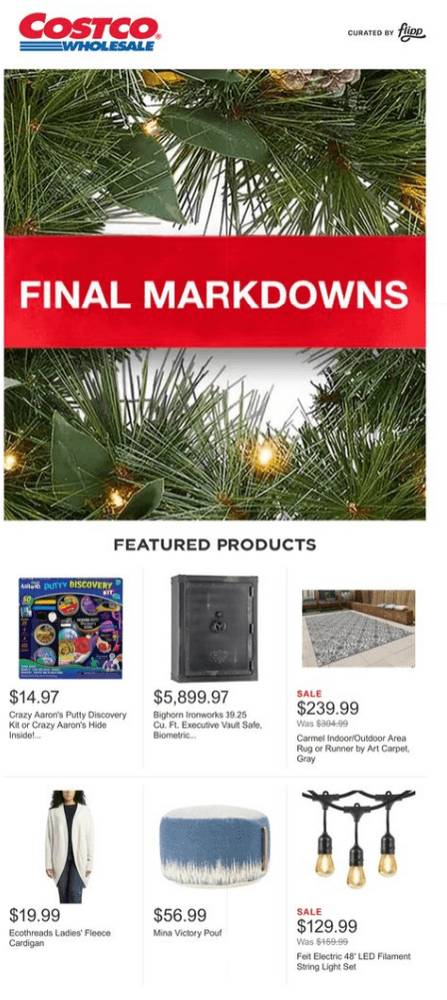Featured on the Costco website, the web page showcases a cheerful and festive design dominated by white, red, and blue color schemes. Prominently displayed is an image of lush green pine needles adorned with bright, twinkling yellow lights, evoking a sense of holiday spirit. Cutting across this image is a bold, red horizontal banner inscribed with "Final Markdowns" in striking white text. Below the festive imagery, the web page highlights various featured products arranged in a well-organized layout. On the left side, there are two rows of products, each row containing three distinct items. On the far left of the second row, a cozy white sweater is featured, with its price clearly marked at $19.99. The overall presentation is engaging and visually appealing, drawing the viewer’s attention to the special offers available.